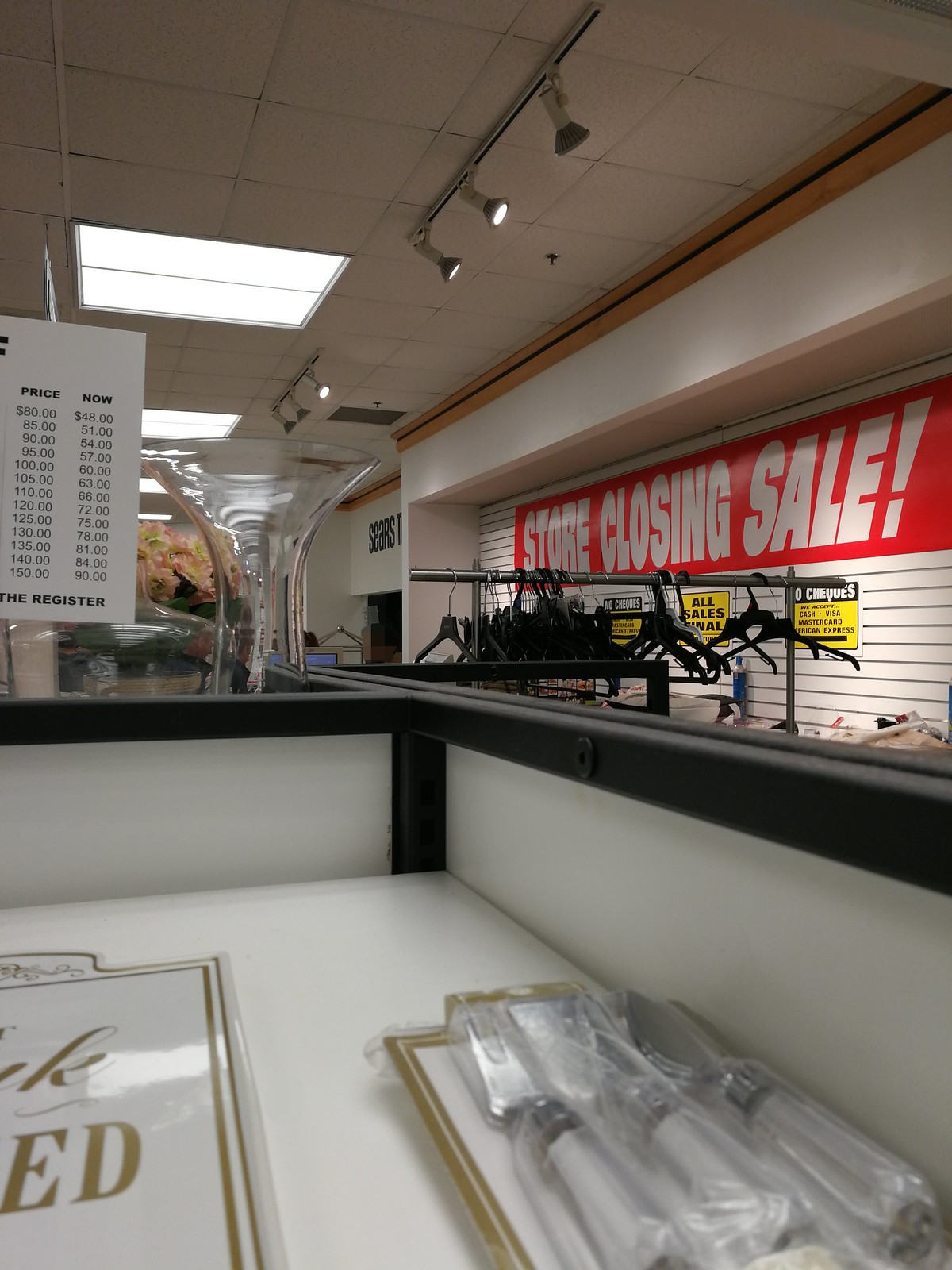The image portrays a forlorn scene inside a store, likely in its final days of operation. The photograph, which is taller than it is wide, captures a desolate retail space devoid of customers. The viewer's perspective is a diagonal glance across the store, resulting in angled lines and a sense of depth. 

To the right, a closed metal grate that resembles a pharmacy window prominently displays a red sign with the words "Store Closing Sale" in bold white letters. Below the sign, an empty rack of hangers evokes a sense of abandonment and finality.

In the foreground, there's the interior of a counter, which features a sign that reads "Objects and Their Wrappers" on its side. The ceiling above is well-lit, showcasing both recessed UV panels and track lighting, contributing to the overall stark and somewhat clinical atmosphere.

On the far wall to the upper left, the remnants of the store's former identity are marked by the iconic "Sears" logo. This confirms that the image is of a Sears store, now in the midst of closing down and clearing out the remaining unsold items. The air of empty aisles and deserted fixtures encapsulates the end of an era for the once-thriving retail giant.